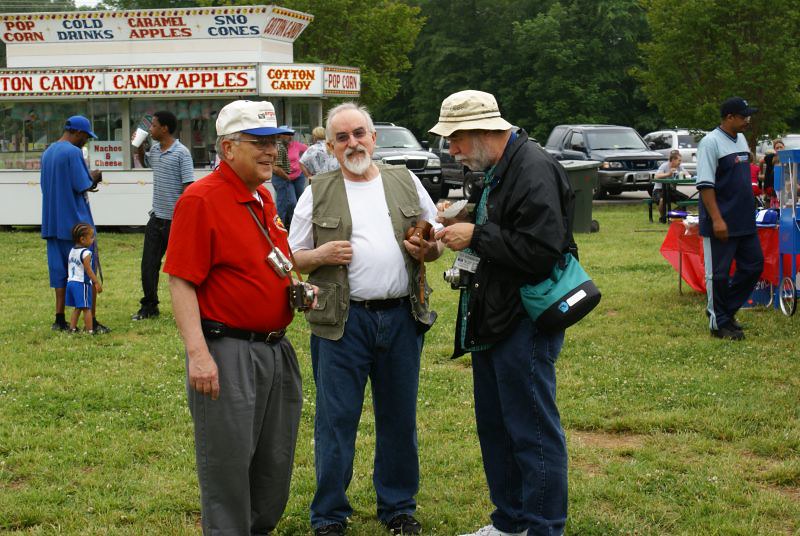The image captures a vibrant outdoor fair or event. At the heart of the scene, three older men are engaged in conversation. The man on the left is wearing a red short-sleeved shirt, a white baseball cap with a blue brim, glasses, and gray long pants. The central figure is dressed in a white t-shirt and a light tan or green vest, has a mustache and a thick goatee, wears sunglasses, blue jeans, and has a camera dangling from his neck. The man on the right sports a black jacket, long blue jeans, and a fisherman's style hat, reminiscent of those worn in "Gilligan's Island," with a camera also around his neck.

Behind them, a bustling parking lot with visible cars includes two black SUVs, a two-door black SUV, and a silver van. In front of the parking lot sits a white food stand with windows on all sides. The stand is adorned with colorful signage: "popcorn" in red, "cold drinks" in blue, "caramel apples" in red, and "snow cones" in blue at the very top. On one side, the words "cotton candy" are visible, and another marquee lists several treats: "cotton candy," "candy apples," "cotton candy," and "popcorn."

In the distance, a solid green tree line frames the scene, providing a peaceful backdrop to the lively affair. Various people can be seen engaged in different activities, including a man holding a child, adding to the friendly and communal atmosphere of the event.